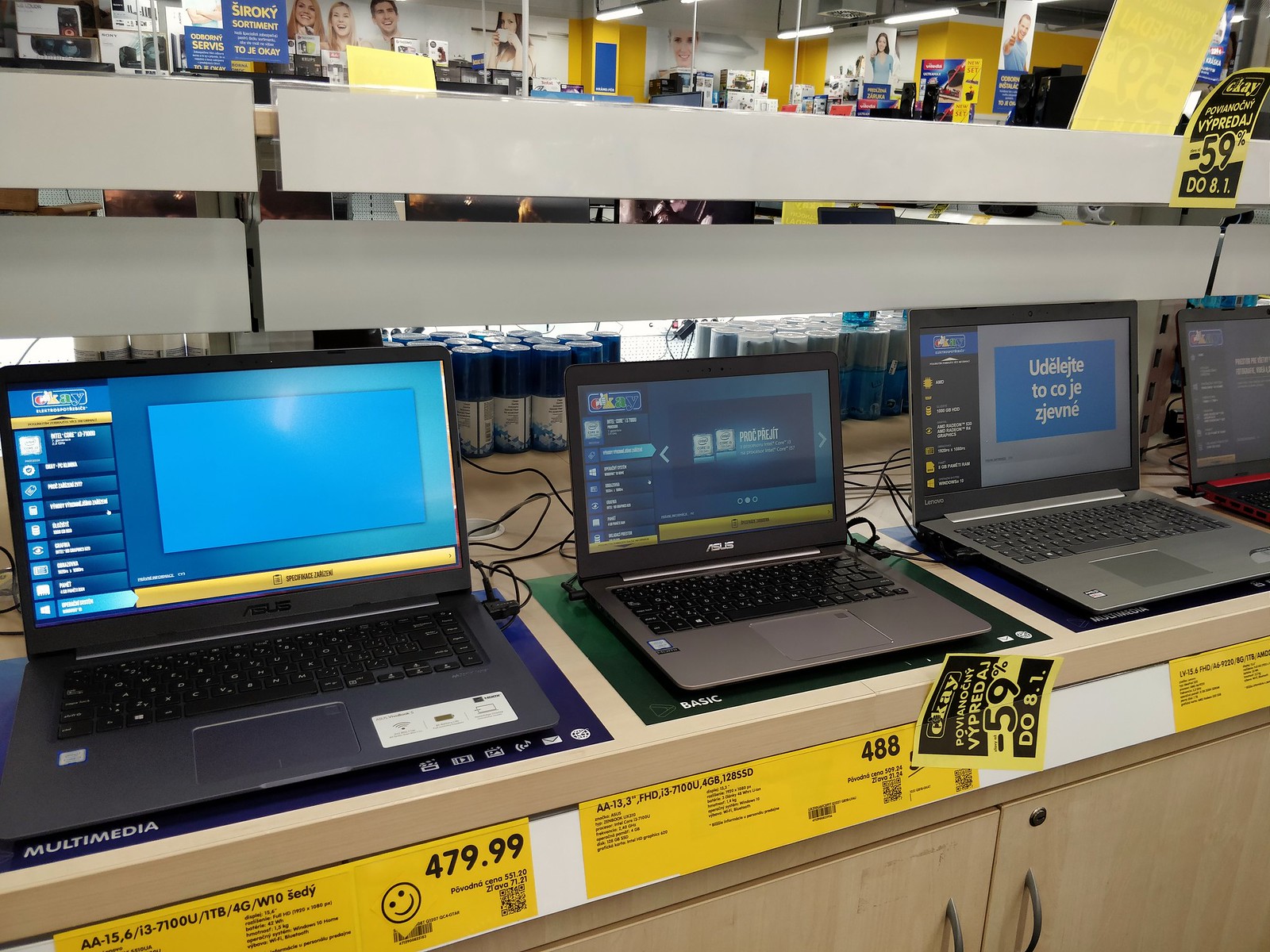The image captures the interior of an electronics store, showcasing a display counter with four laptops. The store's color scheme prominently features yellow and blue, while the countertop is a light-colored wood. Three of the laptops are by Asus, and one is by Lenovo, all with black or dark gray bodies and blue screens. Yellow labels beneath each laptop indicate their price and specifications, with one labeled "Multimedia" and another as "Basic." The background reveals walls adorned with white and yellow patterns, alongside numerous posters of smiling people and electronic gadgets. The store's signage is in a foreign language, possibly Russian or Scandinavian. Behind the laptops, other electronic products are visible, including items for cleaning electronics, further emphasizing the store's diverse inventory. The environment is clearly that of a tech retailer, similar to a Best Buy or Future Shop.